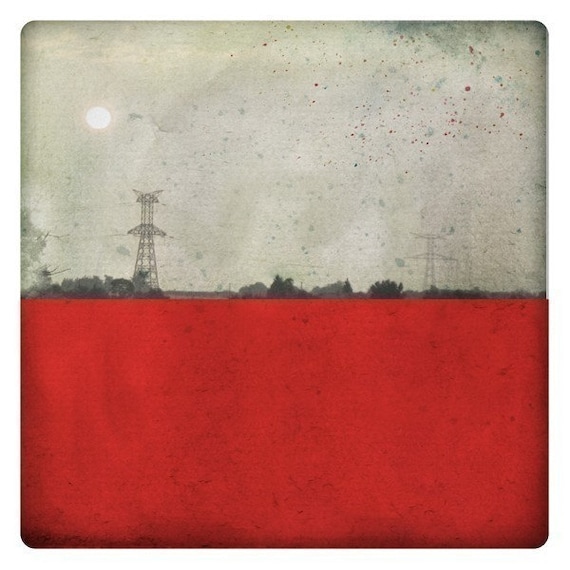This stylized artwork is divided into two distinct sections on a tile-shaped medium with rounded edges and corners. The top half features a black-and-white photograph set against a light grey background, showcasing a sun or moon in the sky. Dominating the scene is a large electrical tower or perhaps a phone tower on the left, extending over the tops of scattered trees and small houses below. The bottom half of the image is a solid, dark red rectangle. Across both halves, random red paint speckles are splashed, imparting a spontaneous, somewhat weathered appearance to the piece.